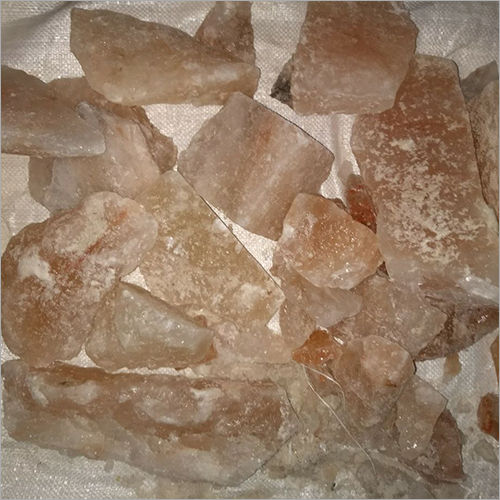The photograph displays an assortment of 12 or so jagged and irregularly shaped crystals scattered across a white tablecloth. The crystals vary in size, with some being larger and others quite small. Their colors range from a light peach or reddish hue to off-white and cream, giving them a somewhat translucent and shiny appearance. The crystals are not uniform in shape, comprising chunks that resemble squares, triangles, and longer forms, all with a somewhat broken or imperfect appearance. The white fabric background accentuates the delicate and varied tones of these unique and scattered crystals.